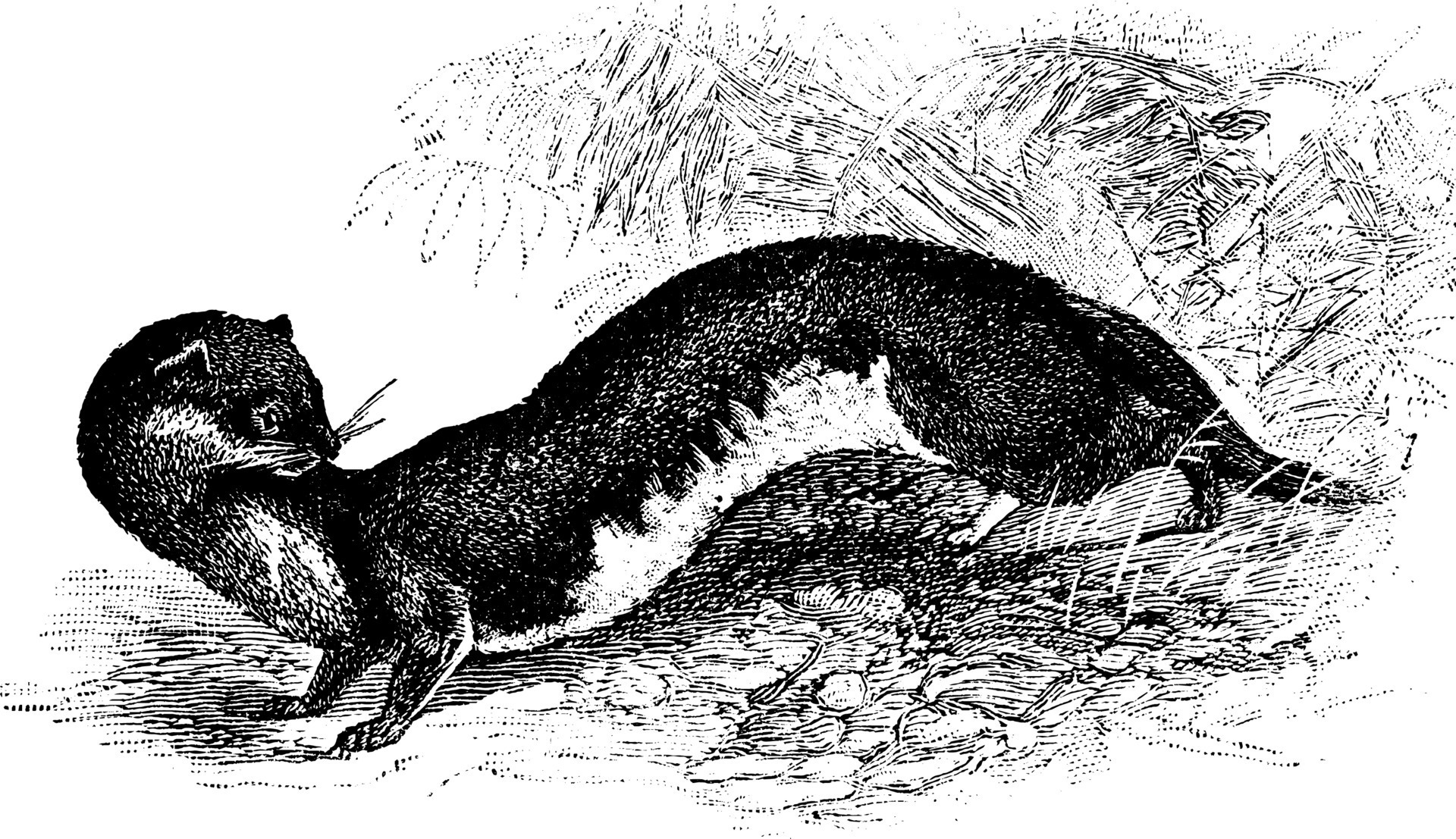This black and white illustration depicts a creature resembling a ferret or possibly a weasel, evoking an old-world charm akin to vintage nature drawings found in books. The creature’s body is notably elongated, with an unusually long neck, suggesting it was drawn from memory with slight inaccuracies. Its black upper body contrasts with a white belly, and it possesses detailed whiskers. The animal is captured in mid-motion, as if pausing to look back over its left shoulder, extending its front paws forward. Emerging from what appears to be bushes or grass, the background remains starkly white, devoid of any text or author credit. Though the creature is intended to be lifelike, it carries an odd sense of disproportion, enhancing the uniqueness of the image. The overall composition is reminiscent of children’s book illustrations, where the detailed yet slightly off-kilter depiction adds a layer of intrigue and nostalgia.